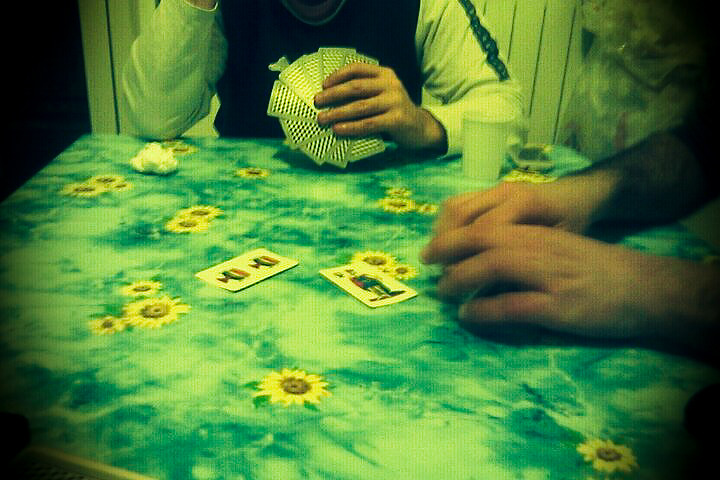The image depicts a table adorned with a green tablecloth patterned with yellow daisies, which, combined with the green filter applied to the picture, gives a distinct greenish hue to the entire scene. On the right side of the image are two men, though their heads are not visible. The man nearest to the center has his hands visible and wears a dark-colored vest over a white long-sleeved shirt. He is holding eight non-standard playing cards, which include unique designs such as a joker or clown-like figure and a chalice. A couple of these cards are also laid out on the table. The other man, positioned further to the right, appears to be holding cards as well, inferred from the way his hands are folded. Between the two men, there is a white cup, possibly containing a beverage, and what looks like a box, likely the container for the playing cards. The setting seems to be indoors, with a white wall featuring blue stripes visible in the background. The overall setup hints at at least two people engaging in a card game, surrounded by a vividly green-tinged atmosphere.